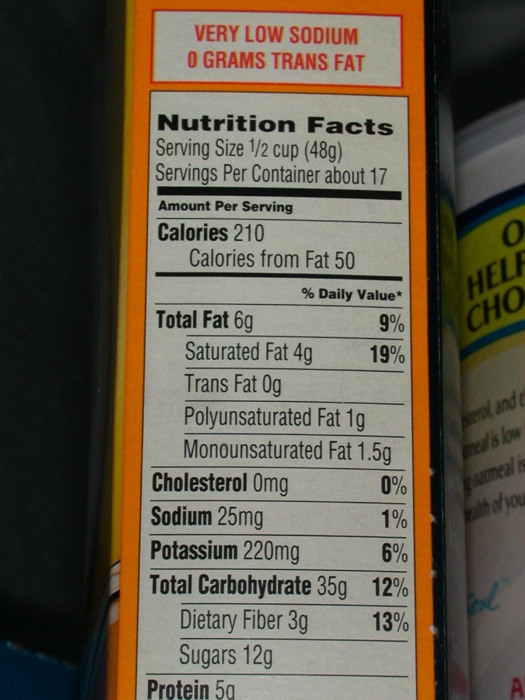This detailed image captures the nutritional label side of a brightly colored orange box, likely for a food item such as cereal. Dominating the top portion of the box, bold orange lettering with a white border prominently states, "Very Low Sodium, Zero Grams Trans Fat." Below this, the nutrition facts panel is displayed on an off-white background with black text. It details that the serving size is half a cup or 48 grams, with 17 servings per container. Each serving contains 210 calories, of which 50 come from fat. The total fat content is 6 grams, including 4 grams of saturated fat, zero grams of trans fat, 1 gram of polyunsaturated fat, and 1.5 grams of monounsaturated fat. The panel also lists percentages for daily values (% DV): total fat is 9%, saturated fat is 19%, cholesterol is 0%, sodium is 1%, potassium is 6%, total carbohydrates are 12%, and dietary fiber is 13%. To the right of the box, partially visible, is another pantry item housed in a cylindrical canister with a clear plastic lid.